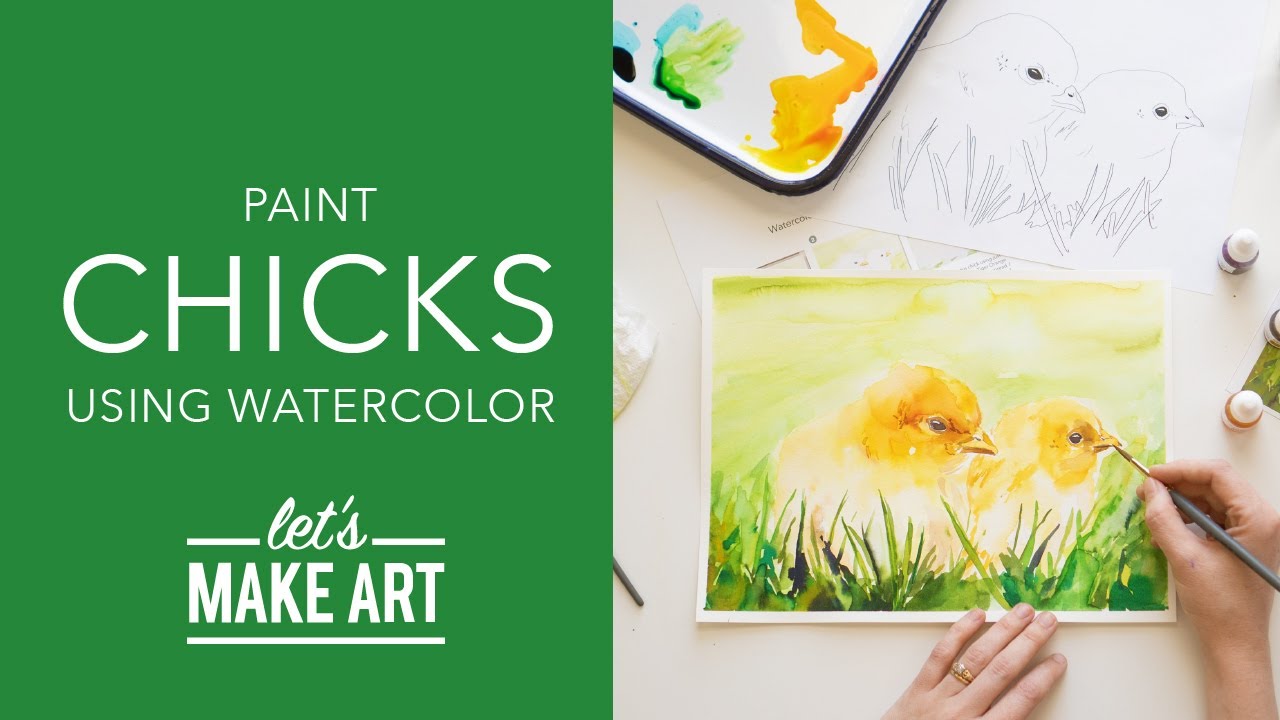The image resembles a postcard for a business promoting a watercolor painting activity. On the left side, set against a green background, bold white text reads "PAINT CHICKS USING WATERCOLORS." In smaller cursive below, it says "Let's make art." The right side of the image depicts a detailed scene where a woman’s hands are visible. Her left hand, adorned with a gold ring, steadies a piece of paper while her right hand, holding a gray brush, paints two baby chicks with golden heads and yellow bodies, set against a backdrop of green grass. Above this live painting, an outlined drawing of two chicks is visible, ready to be painted. The scene includes a paint palette and various paints, all placed on a table, emphasizing the art-making process.